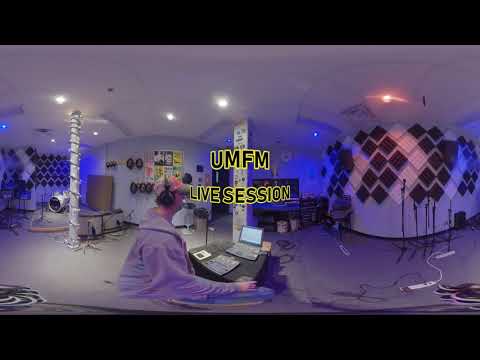The photograph depicts a large studio room with white walls, a white floor, and a white ceiling adorned with small, white lights. The room features several pieces of equipment and decorations, including stickers on the walls and square color patterns in black and white. In the center of the room, there is a person wearing a gray hoodie, a baseball cap, blue jeans, and headphones, seated at a black desk with a laptop and various computer paraphernalia, including a small console. The individual appears to be facing a staged area against the wall, distinguished by the square patterns and equipped with multiple microphone stands. There are numerous cords extending from the floor towards these stands. The image prominently features text that reads "UMFM Live Session" in warped, black, all-caps letters with a yellow outline. Additionally, the studio includes column supports and other equipment such as drums and electrical outlets visible towards the right side of the picture. Blue and red lights add a touch of color to the predominantly white setting.